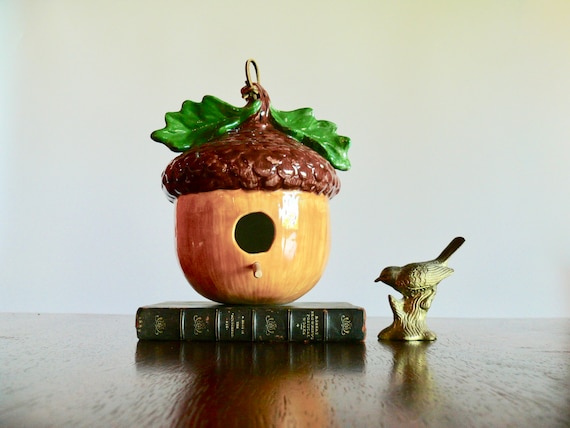In this image, we see a detailed arrangement of ceramic figures placed on a wooden desk with a light gray background. The centerpiece is a ceramic birdhouse designed to resemble an acorn, featuring a light cream-colored brown base and a mottled dark brown cap that mimics the texture of a mushroom. It has two green ceramic leaves at the top and a hole with a small perch beneath it, enhancing its birdhouse appearance. The acorn birdhouse, which is approximately the size of a hardbound book, rests on top of a leather-bound book, anchoring the composition and giving a sense of its scale.

To the right of the birdhouse, there is a small statue of a bird, likely a sparrow, crafted from a metallic material with a golden hue. This bird figurine is not highly detailed, with possibly some subtle shading on the tail. The whole setup is positioned to catch reflections of light, contributing to the aesthetic appeal of the scene. The thoughtful arrangement and the understated color palette create a charming and visually pleasing tableau.